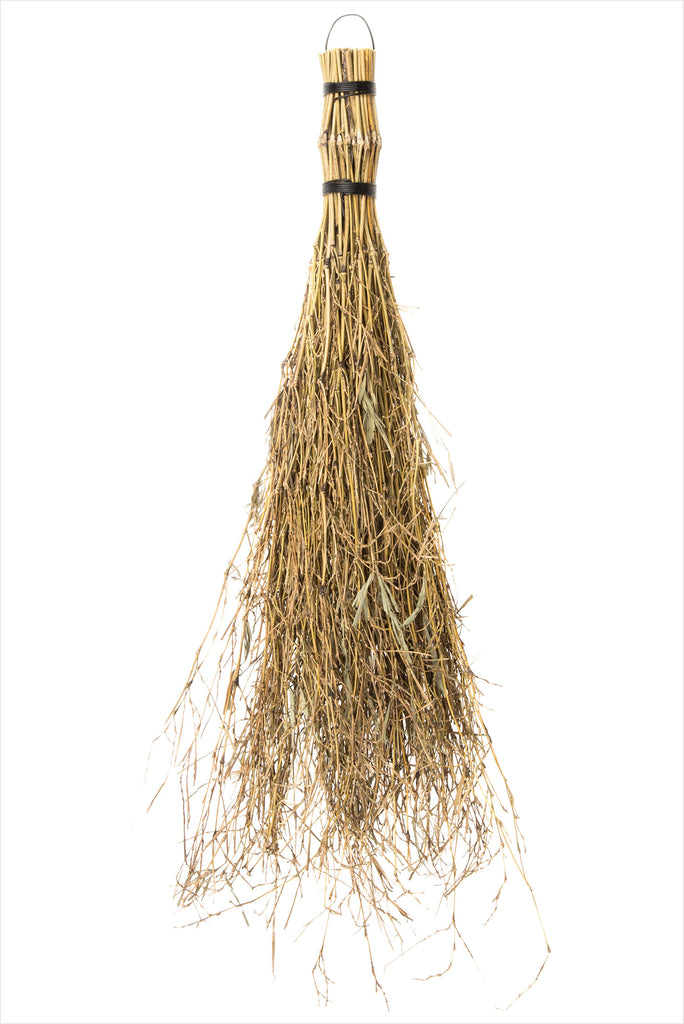The image depicts a hand broom comprising several dried plant strands, possibly straw, that are tightly bound together near the top with two black bands. A small loop, which looks like a cord or metal, is present at the top, likely intended for hanging the broom. The plant material, mostly in shades of brown and tan, fans out messily at the bottom in a bristly, cone-like shape, giving the appearance of the broom's sweeping end. Despite the plain white background providing no scale reference, the broom feels fairly large and robust, yet the texture of the straw, interspersed with a few dried leaves, suggests it might be brittle and prone to breaking. Encased in a clean, grayish border, the image accentuates the natural, somewhat rustic aesthetic of the broom, which lacks a traditional long handle, making it necessary to bend down for use.